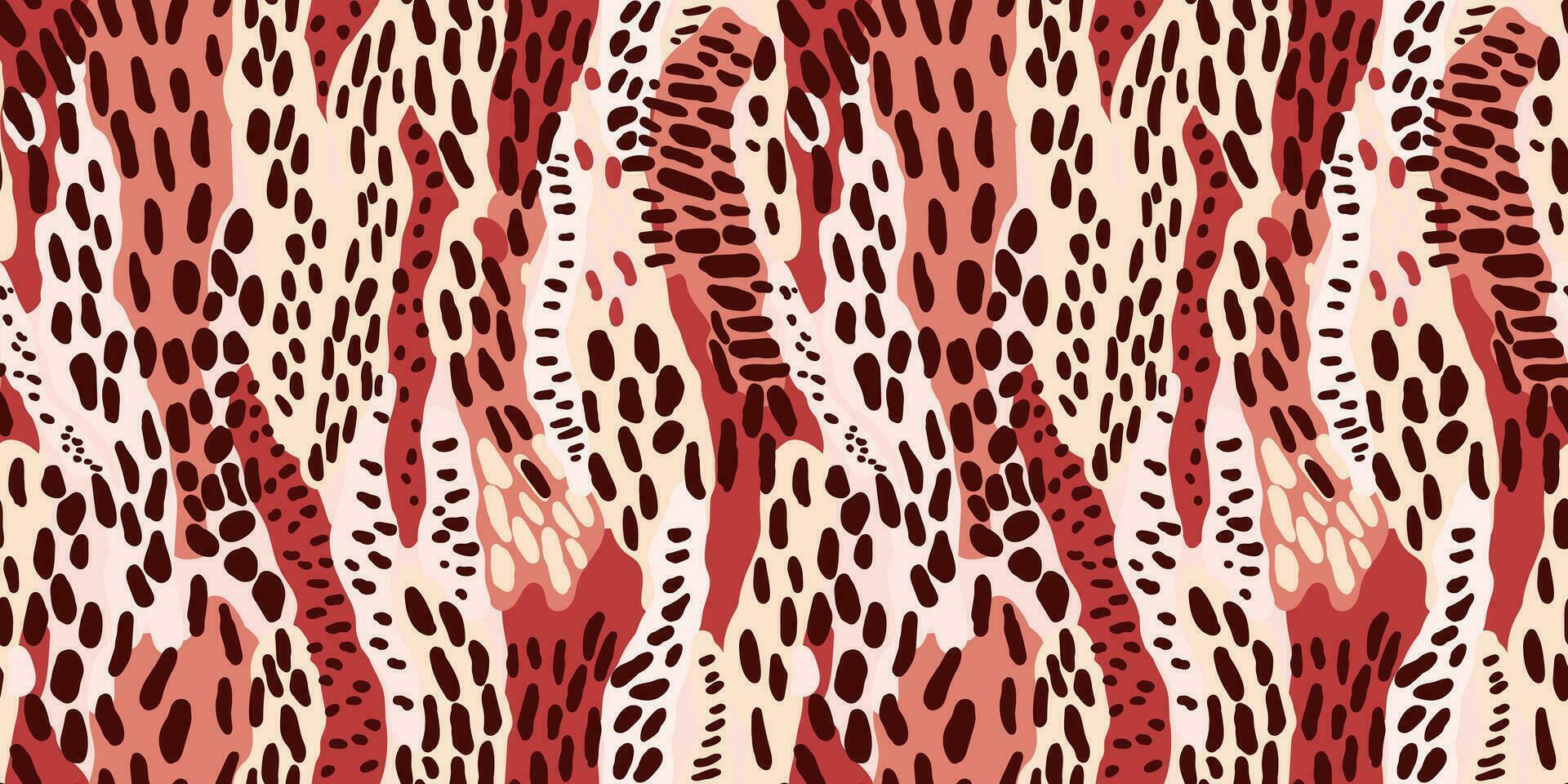The image is an abstract, contemporary piece showcasing a complex pattern that evokes an animal print, resembling giraffe or leopard spots. The composition features a chaotic blend of various shapes and colors. Numerous irregular circles and oval spots in black, varying in size, are scattered uniformly across the design. These spots overlay abstract, banded regions that fluctuate between deeper red hues and lighter watermelon pink tones. Additional elements include zigzag zebra stripe-like shapes that traverse the top and bottom of the image, interspersed with lighter shades of yellow and white. The overall effect is a richly textured, spotted canvas, suggesting random splashes of paint with no discernible subject, embodying the essence of modern abstract art.